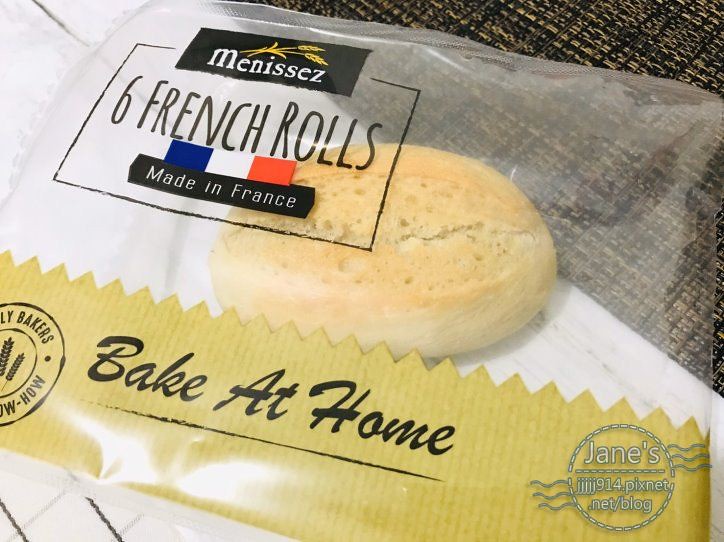The image depicts a clear plastic bag containing a single French roll, lying on a surface that has a white area and a section with black and tan-colored cloth. The packaging displays a logo at the top that reads "MENISSEZ" in a black rectangle, accompanied by a yellow wheat or barley illustration. Below the logo, it states "Six French Rolls" with a partial blue, white, and red design representing the French flag alongside the text "Made in France." A prominent gold spiked bar stretches across the bag with the words "Bake at Home" in black. Additionally, on the right side of the bag, there is a white circle containing the text "James JJJJJ914.pixnet.net/blog," indicating a source or reference.